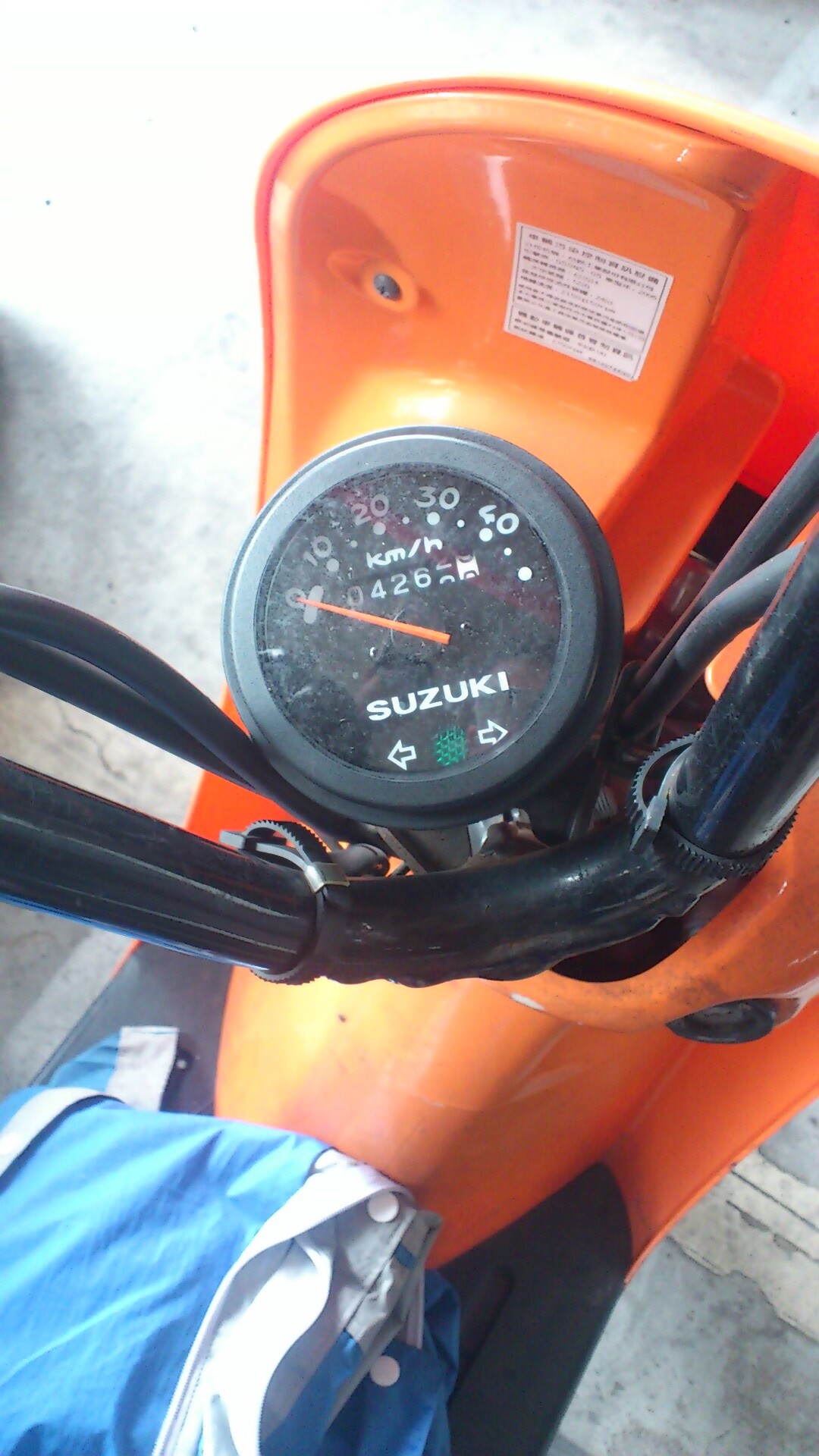This color photograph, taken in a garage with a concrete floor, provides an intimate, zoomed-in view of a Suzuki dirt bike's odometer. The odometer, which displays zero and has an orange needle, is framed by the handlebar's base and other instrument lights. The numbers on the odometer dial, reaching up to 40, are written in white, as is the Suzuki branding. There is a green light located below the word "Suzuki," flanked by indicators for both left and right turn signals. The odometer shows a total of 426 miles. An obscured manufacturer's sticker is visible above the odometer. A person wearing a blue shirt sits on the orange and black dirt bike.